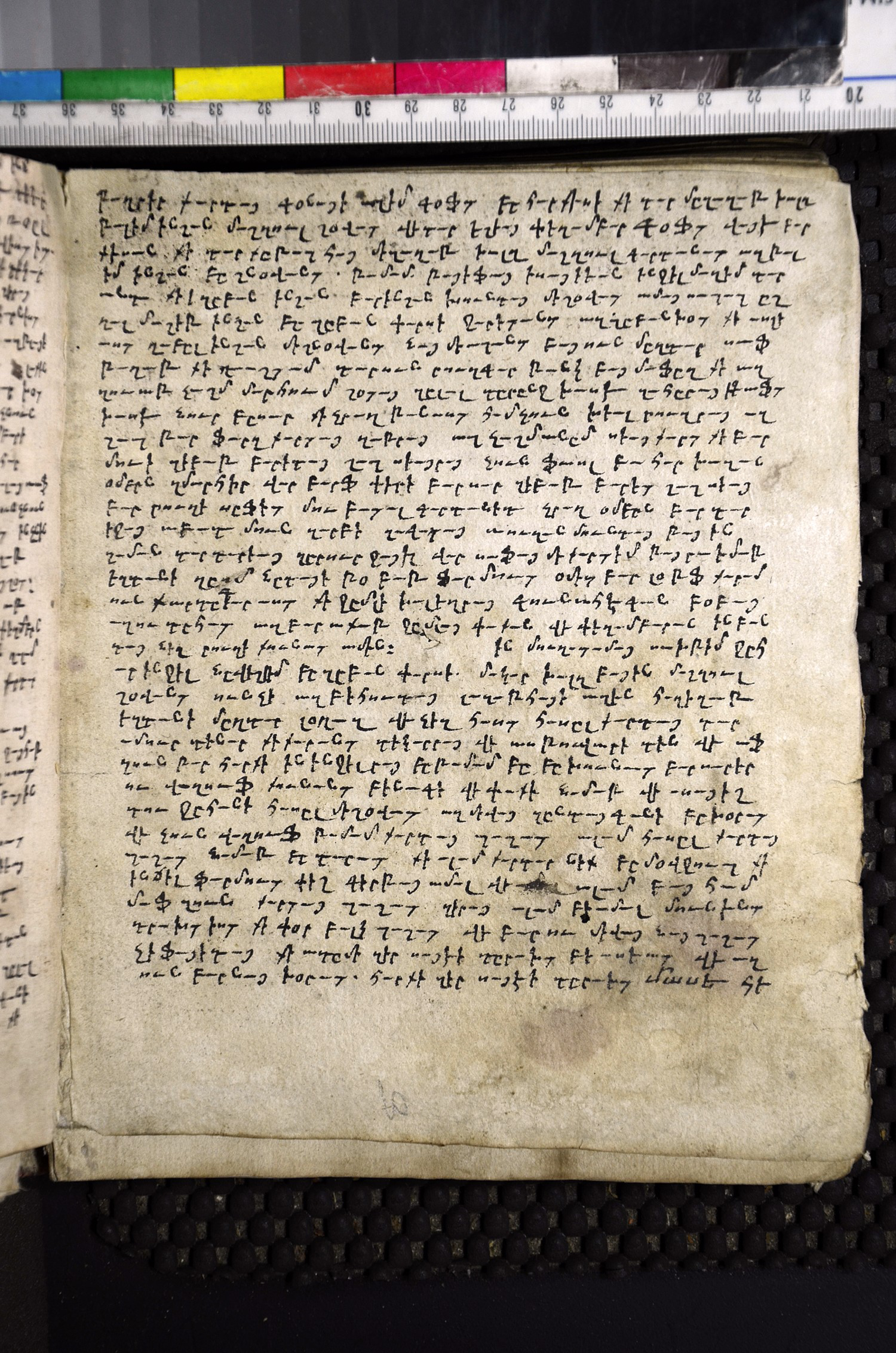The photograph captures a venerable, centuries-old book with pages that exhibit considerable wear and aging, featuring brownish, yellowish edges that suggest significant antiquity. The page predominantly visible in the center of the image is adorned with handwritten text in an indecipherable script that some have likened to Arabic or similar Middle Eastern languages, characterized by ornate and intricate lines. The ruler, positioned along the top edge of the book, appears to be a white measuring tool marked from 20 to 37 centimeters, indicating the page is around 17 centimeters wide. Above the ruler, there are colored blocks in a sequence of blue, green, yellow, red, orange, pink, white, grey, and black, likely for color calibration or documentation purposes. The page itself seems to be documented in a controlled setting, possibly within a museum or archival repository, with a black computer keyboard partially visible at the bottom of the image against the dark background. The overall scene suggests a meticulous effort to catalog and preserve the ancient manuscript.